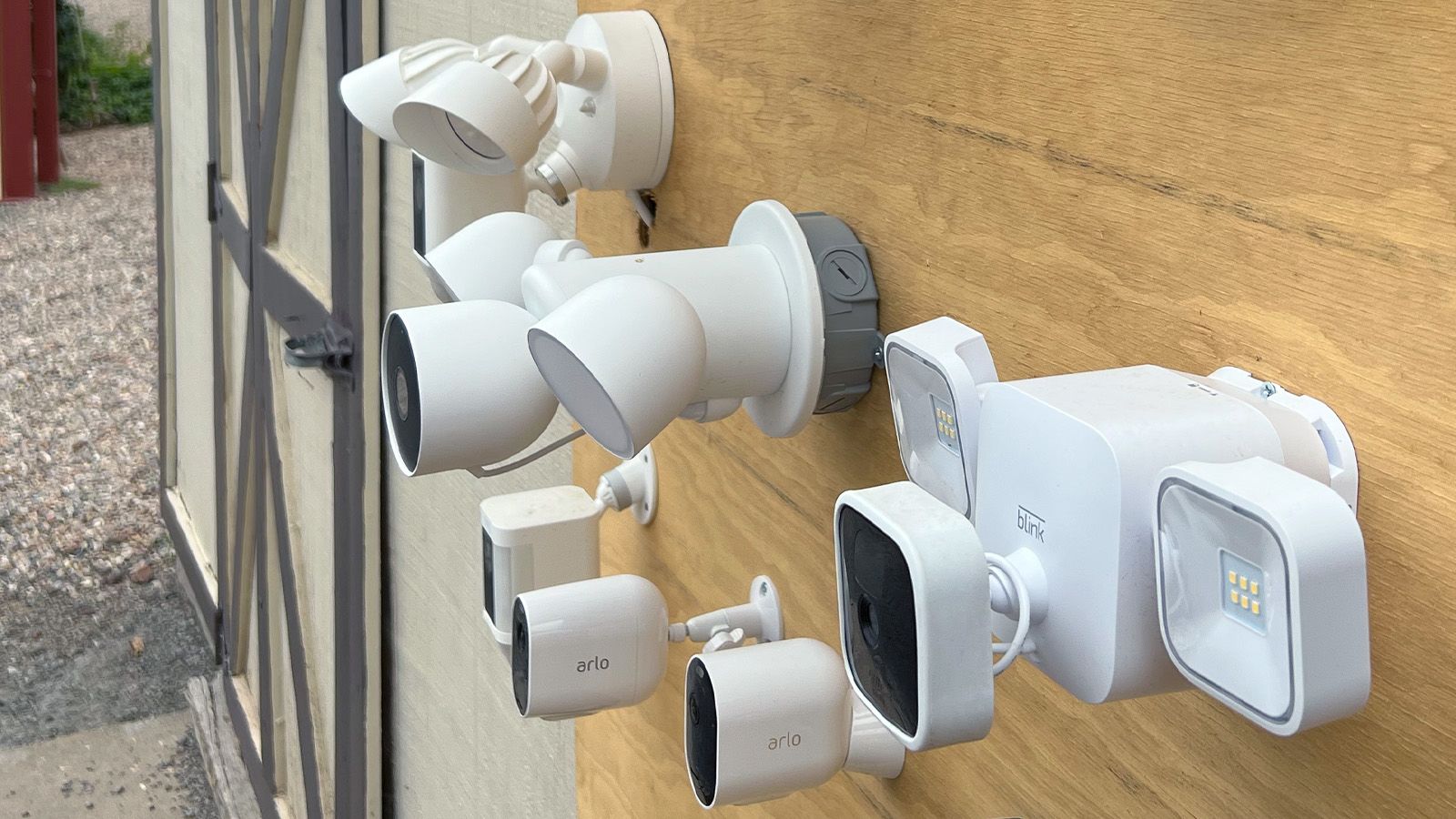This close-up photograph features the exterior of a wooden shed, showcasing a collection of outdoor security devices and lighting fixtures attached to a large piece of plywood on the shed's wall. The shed's facade includes a gray and cream-colored door, and it is situated on a bed of gravel. In the background, red posts and lush greenery add context to the setting.

The focal point of the image is the array of security devices and lights affixed to the plywood. The plywood is brown, contrasting with the shed's other wooden components which are white and gray. The devices are predominantly white, with black and gray accents, and include LED lights with rectangular sensors, as well as various cameras. Notable brands visible on the devices include Aria, Arlo, and Blink. The Blink device is distinctive with its three square appendages, while the Arlo labels are primarily on the motion sensor cameras.

One of the lighting fixtures, positioned above the rest, stands out as an older model and features two spotlights in white. All the devices, despite their different shapes and sizes—ranging from rectangular to round—are currently powered off, indicating they are inactive in the photo. This detailed assembly suggests a comprehensive security system intended for monitoring the shed's vicinity.